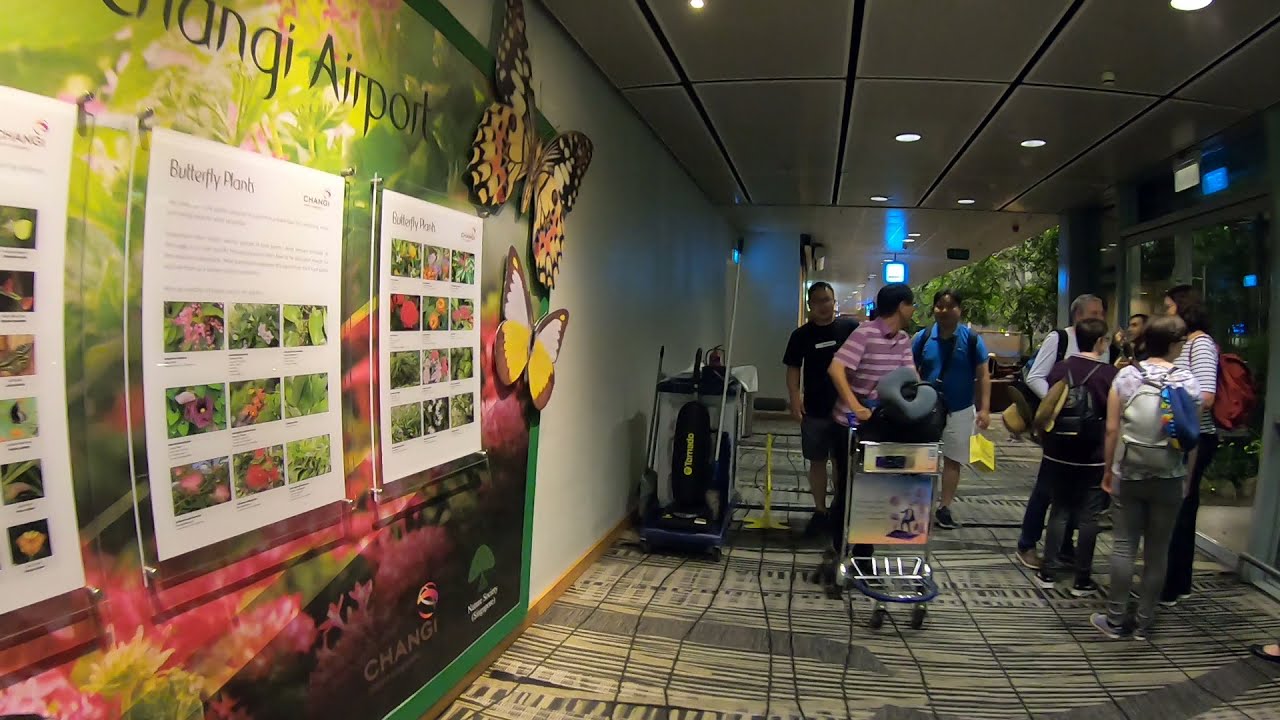The image depicts a bustling indoor scene set in what appears to be an airport terminal, probably named Shangyi or Chengyi Airport, although the sign's first word is unclear. Prominently displayed on the left-hand side is a large, colorful mural featuring flowers and two big butterflies. Below this mural are several smaller posters showcasing various types of butterfly plants in different colors. The mural and posters together create an attractive, vibrant display dedicated to butterfly plants.

Adjacent to this display is a white wall, and the black, gray, and cream-colored rug on the floor indicates the terminal's décor. Various groups of people are visible throughout the scene. On the left, an Asian family visibly maneuvers carts loaded with luggage. In contrast, on the right side, a mixed group of individuals, likely a family, is gathered and conversing while holding backpacks. This group includes a man with gray hair dressed in a white shirt and jeans, a woman in a striped shirt with a red backpack, and two young individuals—one with short hair and glasses, wearing gray pants, and the other possibly a young man or woman with short hair and a backpack. This diverse collection of travelers appears to be waiting for their flight near what seems to be a store. The ceiling and floor details and the general busyness further reinforce the setting as a typical airport terminal.